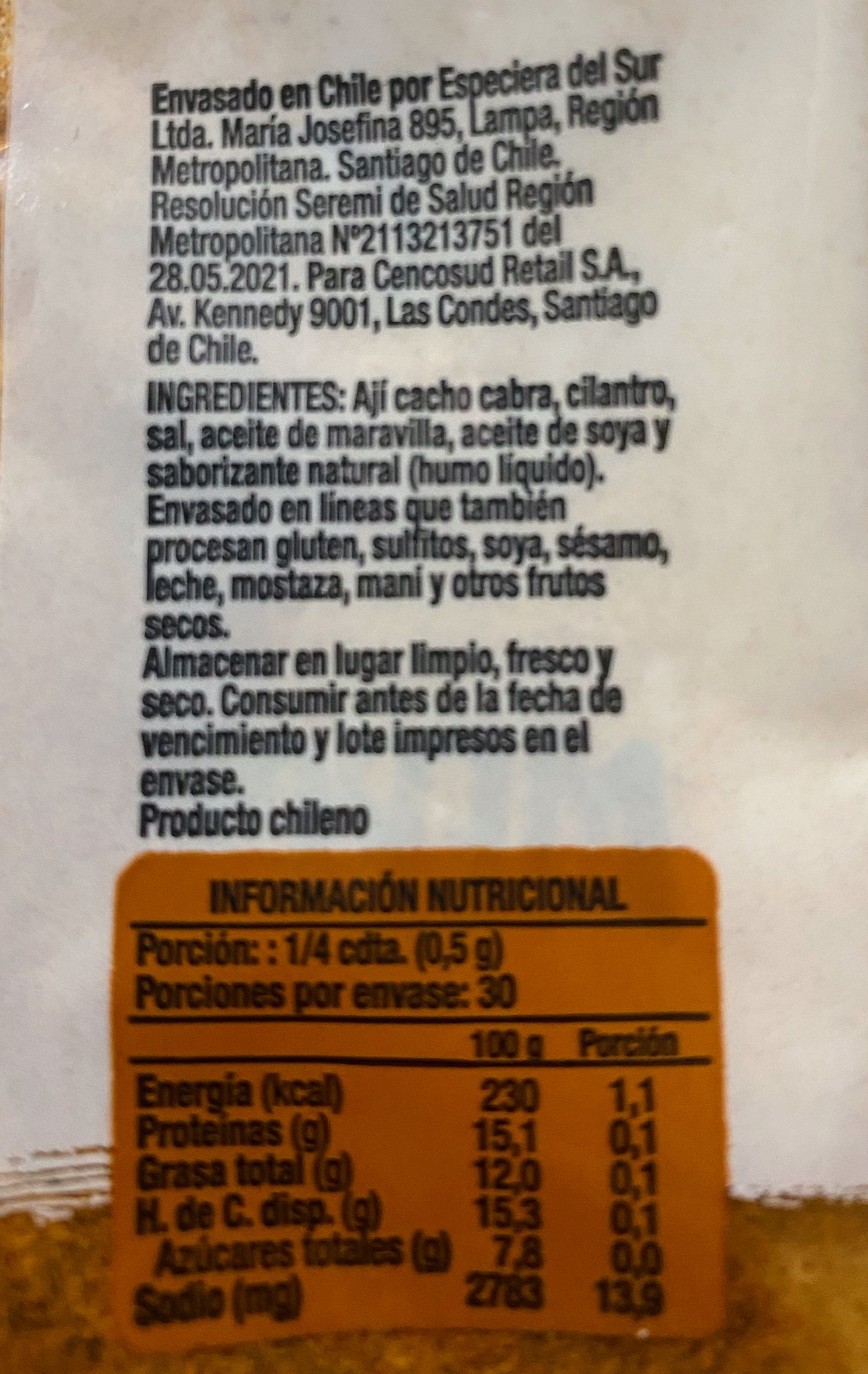The image showcases the backside of a food product packaging. The wrapper is predominantly white, with a segment at the bottom featuring a light, grainy yellow color. The upper portion of the packaging is adorned with a list of ingredients and directions, which are written in a foreign language. The lower section contains a distinct light brown colored square compartment that houses nutritional information. This section meticulously details the contents of the food product, listing proteins, fat, sodium, and calories in both grams and percentage values.